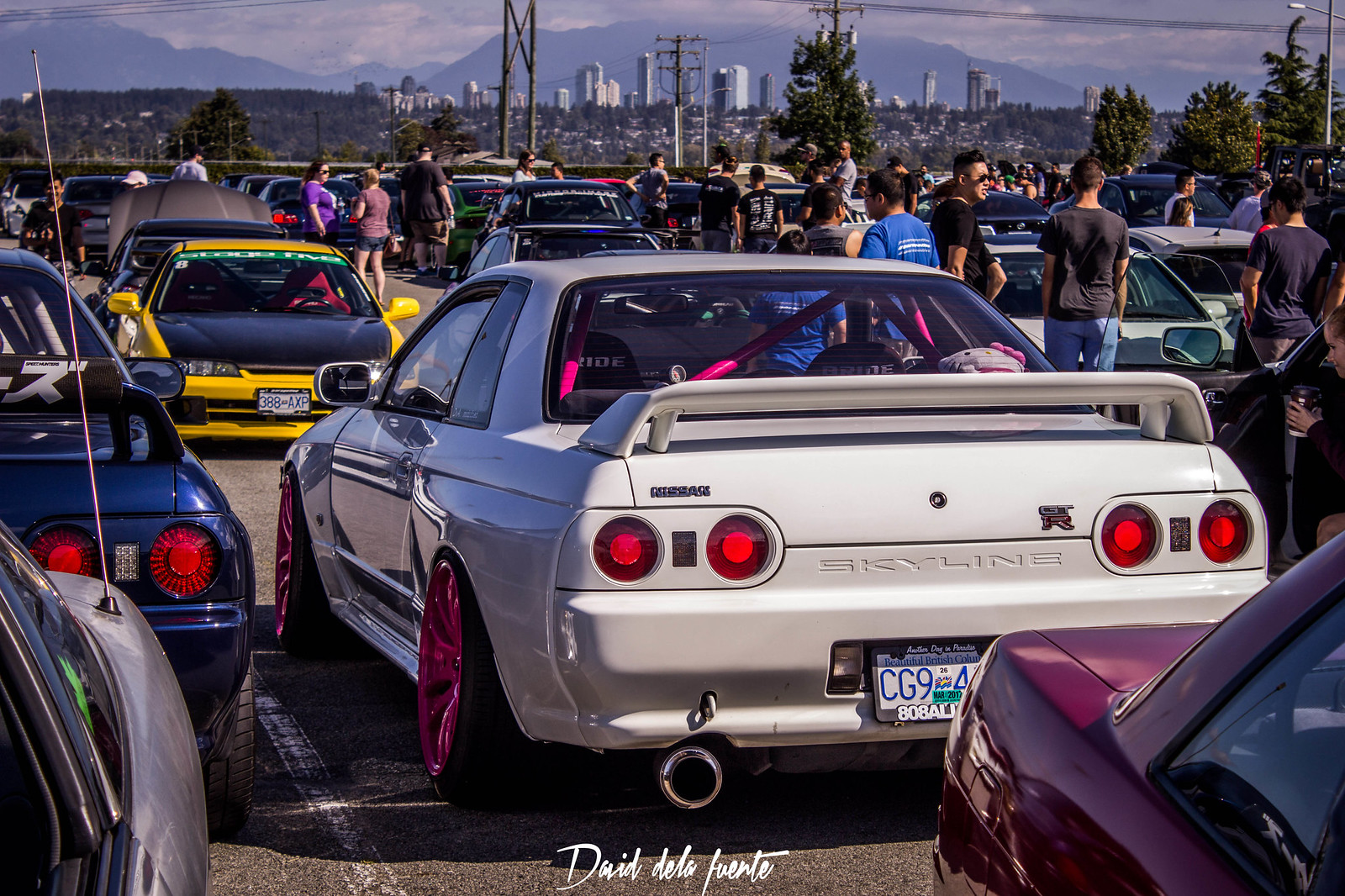The image captures a vibrant outdoor car meet, prominently featuring a white Nissan Skyline GT-R with pink rims and a large exhaust tip, clearly labeled "Skyline" on its rear bumper. This car is the focal point, alongside a similar blue Nissan Skyline. The scene unfolds in a spacious parking lot, bustling with numerous cars and people—mostly men with a few women—enjoying a sunny, partly cloudy day. The event appears to be a gathering for sport or muscle car enthusiasts in British Columbia, as suggested by the visible license plates. The background showcases a detailed city skyline set against a distant mountain range and dotted with light poles, power lines, and a few trees, enhancing the picturesque view. This engaging moment, captured during the daytime, adds a layer of authenticity with a name subtly noted at the bottom of the photo.